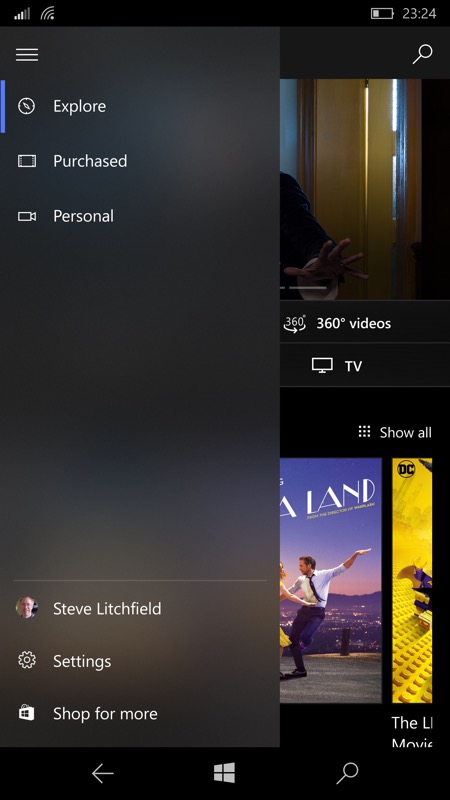In the image, a user appears to be navigating a digital movie purchasing platform. The interface displays several movie titles prominently, including "La La Land," which is partly obscured by other elements. Also visible is another, partially cut-off, movie titled "Lego Land" to the right. The screen's background is black, creating a sharp contrast with the white text and icons.

In the top bar, military time is shown as 23:24, alongside battery life and a Wi-Fi signal indicator on the left. There's a horizontal menu below the time, featuring options such as "Explore," "Purchase," and "Personal," all highlighted in white due to the dark theme. Below this menu are detailed account options, including user "Steve Litchfield" signed into the movie account, a gear icon for settings, and a "shop for more" button. Navigation icons like a back arrow, a Windows logo, and a search icon are also present.

The image appears to be partially cut off at the top, showing a scene from an unidentified movie where a person is sitting at a table near a window with blinds. A "360-degree videos" section with a TV icon is also visible. Overall, the interface is neatly organized, with a show-all button to help users explore more movie options.